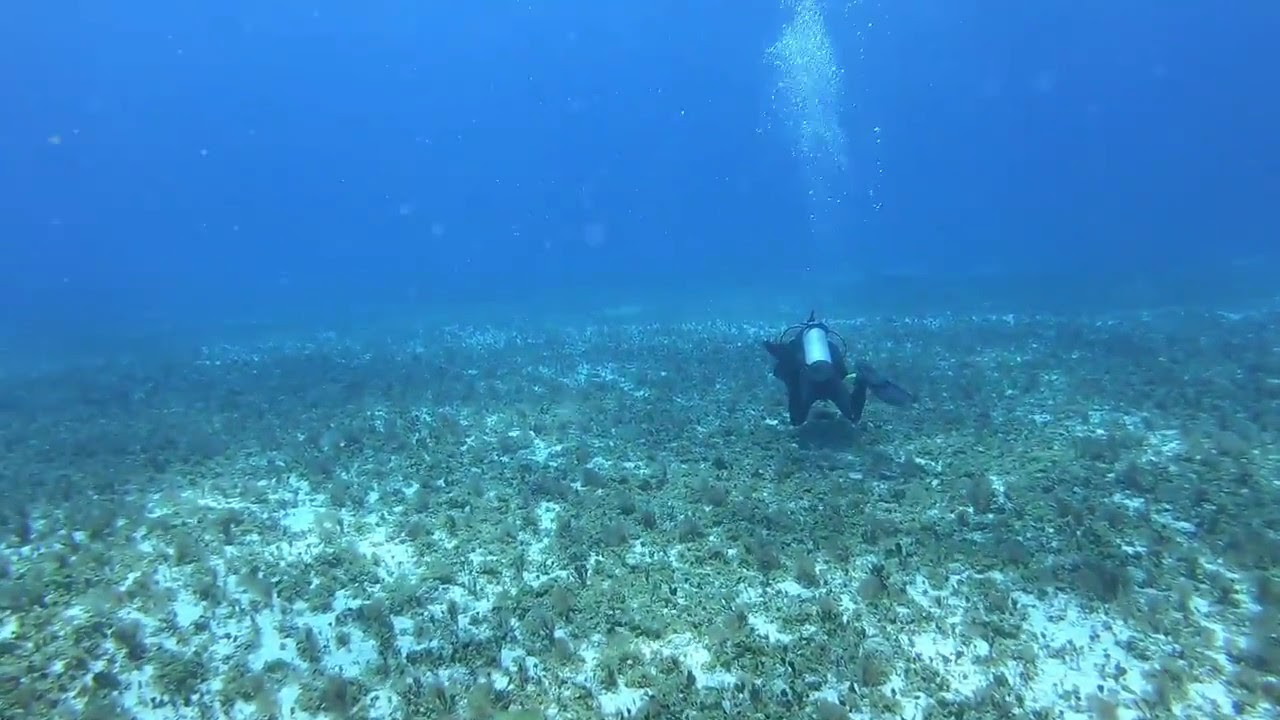The underwater photograph captures a scuba diver swimming slightly to the right of center, facing away from the camera. Wearing an all-black diving suit, fins, and a silver oxygen tank, the diver glides near the sandy seafloor, which is a mix of white sand dotted with numerous green plants, possibly seaweed or coral. Rising from the diver's tank, a stream of bubbles ascends towards a vast blue expanse above. Small rocks and faint white dots—potentially debris or distant fish—pepper the background, adding to the serene yet mysterious underwater landscape. The clear water allows for a detailed view of the diver and the aquatic environment, with the seafloor vanishing into the deep blue distance.